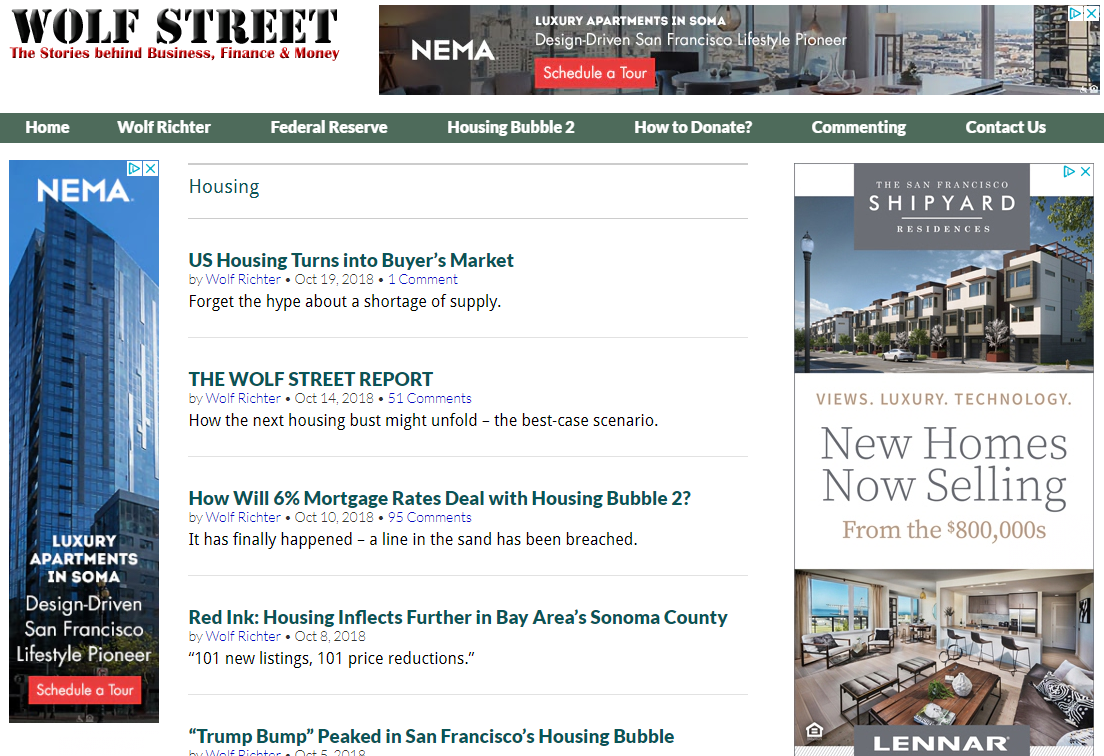The image is a screenshot from the Wolf Street website, which focuses on insightful stories related to business, finance, and money. The top left corner prominently displays "Wolf Street" alongside its tagline "The stories behind business, finance, and money."

A high-resolution banner image spans the top, capturing a breathtaking view from a high-rise, possibly a luxury apartment or office building. Overlaying this image, text promotes "NEMA Luxury Apartments in SoMa," highlighting its design-driven approach and unique San Francisco lifestyle. A striking red button invites users to schedule a tour.

Below the banner, a green navigation bar lists categories: Home, Wolf Richter, Federal Reserve, Housing Bubble 2, How to Donate, Commenting, and Contact Us.

The main content area is dedicated to housing news, featuring several article links: "U.S. Housing Turns into Buyer's Market," "The Wolf Street Report," "How Will 6% Mortgage Rates Deal with Housing Bubble 2," "Red Ink Housing Inflects Further in Bay Area, Sonoma County," and "Trump Bump Peaked in San Francisco's Housing Bubble."

On the left side, an image of a luxurious apartment building is accompanied by another "Schedule a Tour" button. The right side features an advertisement for "The San Francisco Shipyard Residences," showcasing images of upscale condos. It emphasizes views, luxury, and advanced technology, with homes starting from the $800,000s. The ad is from Lenar.